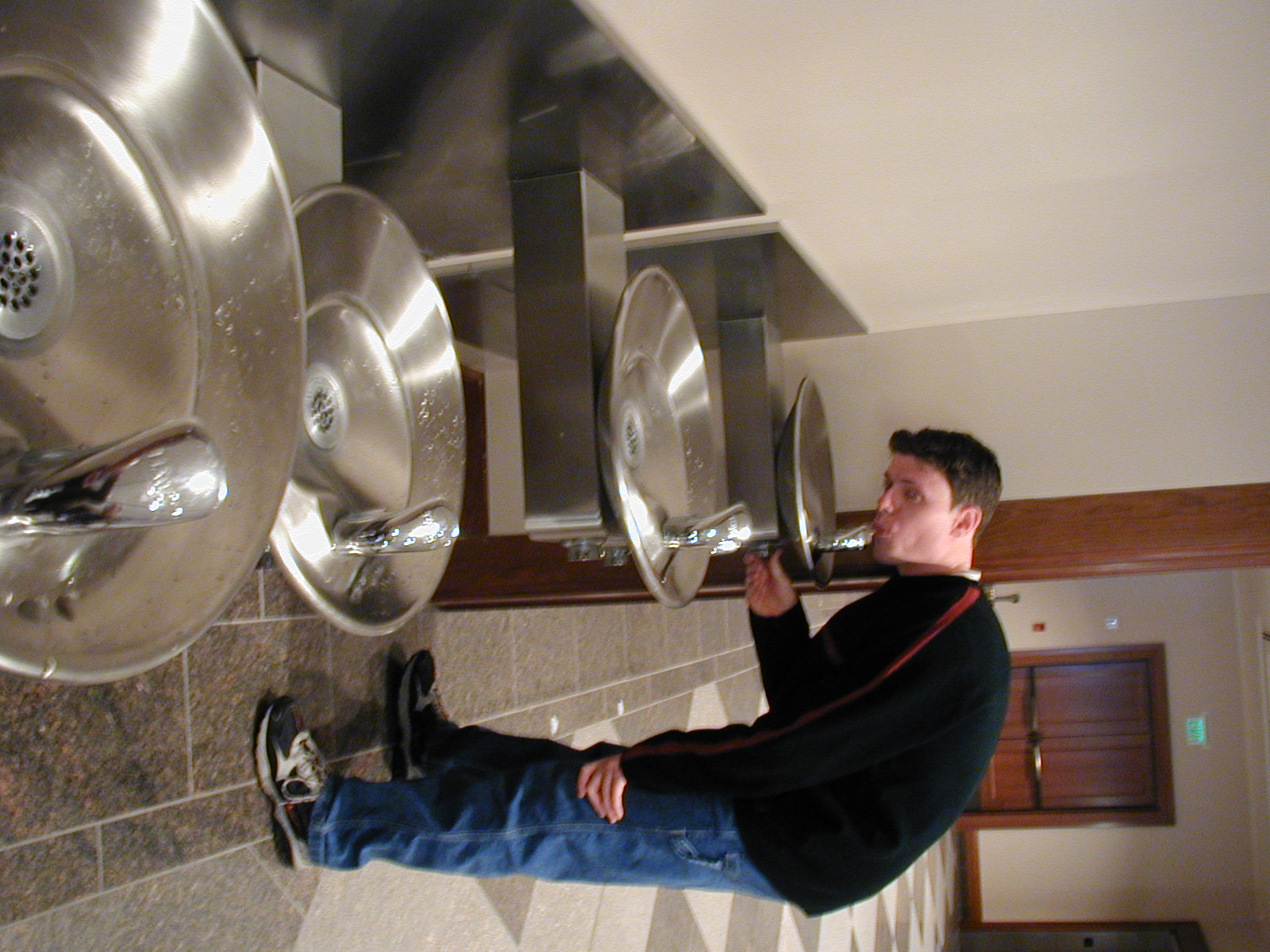The image depicts the interior of a bathroom with its orientation seemingly rotated 90 degrees to the left. Dominating the scene are four water fountains, each featuring silver metal plates paired with brass or polished silver basins perforated with drain holes. The background reveals off-white walls and dark brown, shimmering columns flanking a set of brown doors enclosed within brown frames. The flooring is a combination of brownish-grey marble. Nestled against this backdrop, a person is captured mid-drink at the first fountain. The individual, sporting a black sweater with red stripes, blue jeans, and brown-and-white running shoes, stands out with their white complexion and brown hair. Despite the unusual angle of the photo, which makes the person appear horizontal relative to the frame, the detailed elements of the bathroom fixtures and attire of the person are vividly discernible.